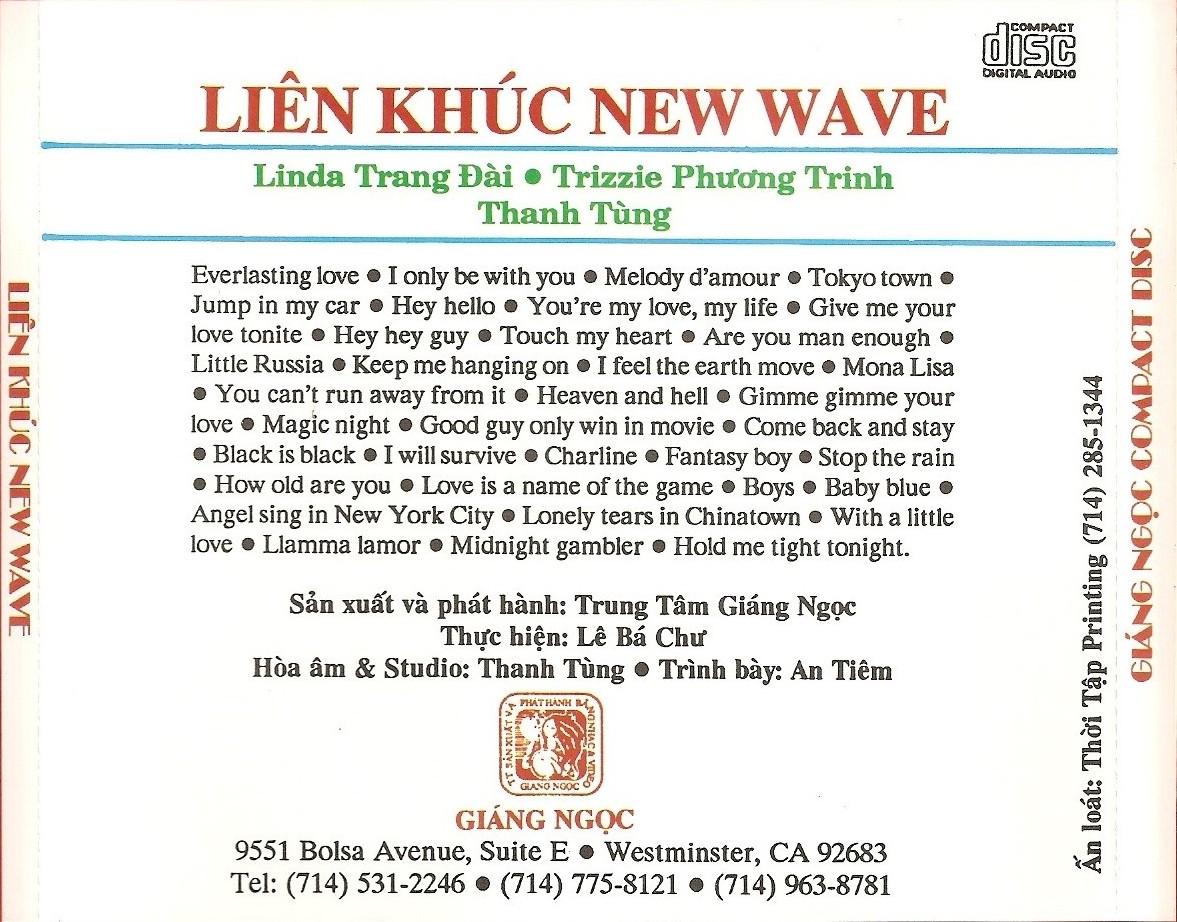This image appears to be the back of a CD case with a well-defined design and textual layout. The background is completely white with a slightly faded look. In the top right corner, there is a small box that reads "Compact Disc Digital Audio," which is a common label on CD cases. At the top of the cover, in bold red capital letters, it says "LIEN KHUC NEW WAVE." Below this title, several names are listed in green text: Linda Trang Dai, Trizzy Fung Trinh, and Tan Tang. 

Lower on the cover, there is a comprehensive list of track titles in black text, some with filled circles separating them. The track listings include songs such as "Everlasting Love," "I'll Only Be With You," "Melody D'Amour," and "Tokyo Town" among many others. Beneath the song titles, there appears to be text in a different language followed by a red logo. Finally, at the very bottom in black text, there is an address accompanied by three telephone numbers.